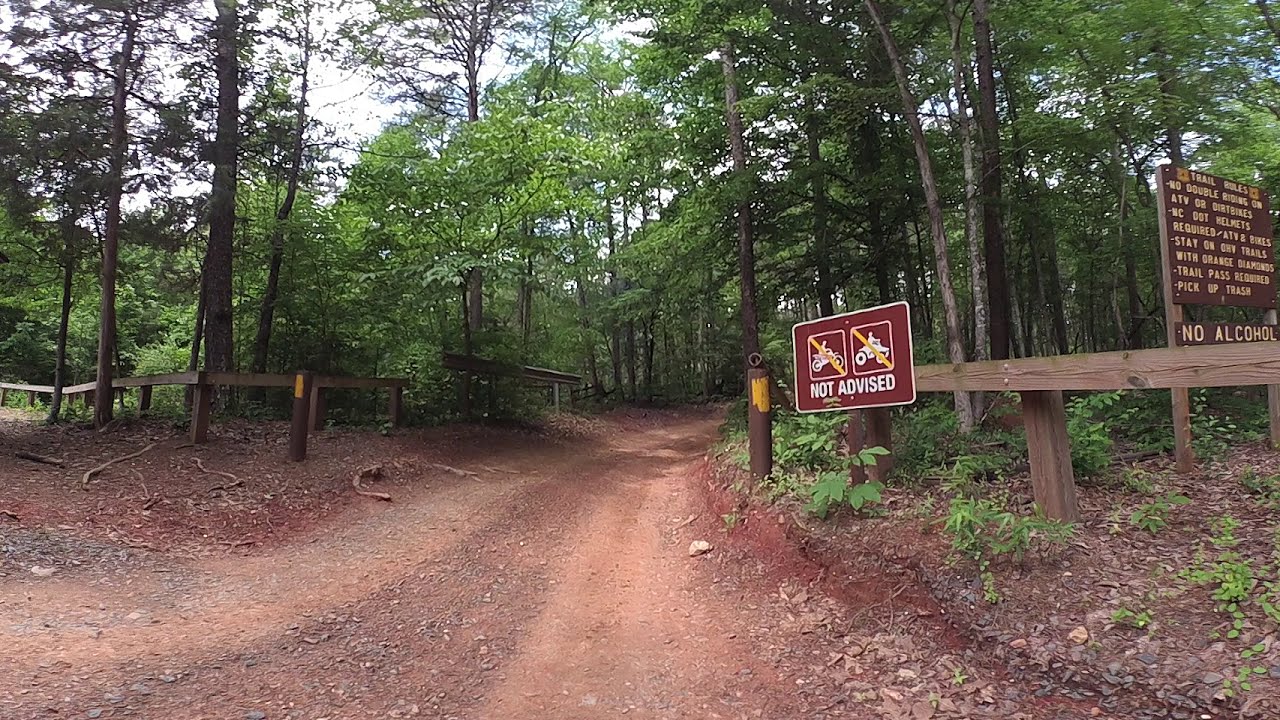This outdoor image features a dirt road winding through a densely wooded area, surrounded by tall trees whose leafy canopies obscure much of the sky. The road, framed by simple wooden fences on both sides, stretches from the bottom edge of the image towards the center. The various shades of brown, red, yellow, white, green, tan, and gray dominate the scene, emphasizing the natural setting and the day’s clear sky.

On the right side of the road, there is a brown trail sign prominently displaying the trail rules, including prohibitions against double riding on ATVs or dirt bikes, stating no DOT helmets required, ATVs are to stay on trails marked with orange diamonds, a trail pass is necessary, and reminders to pick up trash and abstain from alcohol. Although the text on the sign is small, these critical guidelines are readable. Further down, there's another smaller maroon sign with a white outline and a yellow crossed-out symbol indicating that bikes and mopeds are not advised.

The image conveys serenity and solitude, with no visible people, structures, or animals, emphasizing the untouched natural beauty of the mid-forest trail.